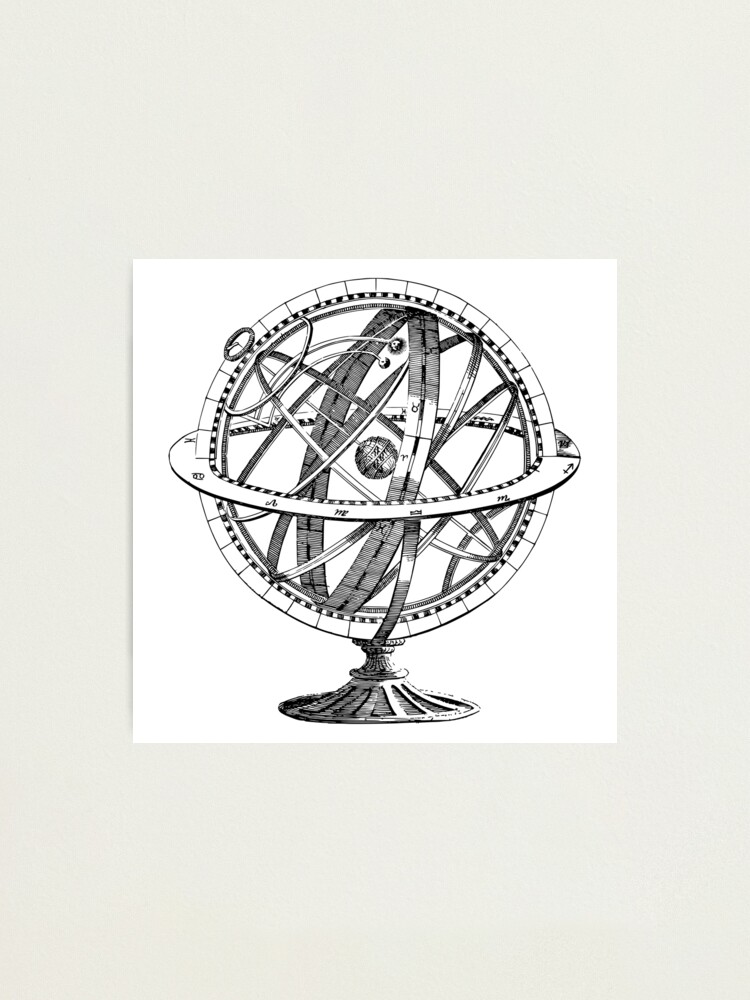This is a detailed pencil drawing depicting an intricate, cylindrical globe-like structure, primarily rendered in black and white. The image showcases multiple concentric circles intersecting and connected, each adorned with meticulous measurements. At the core lies a solitary solid circle, potentially representing Earth or the Sun, surrounded by approximately eight other non-solid, interlinked circles. The circles span various directions, creating a complex, multidimensional appearance. The entire structure is mounted on a stand, with delicate metal frames, adding a touch of realism despite its hand-drawn nature. The drawing sits against a stark white square background, which itself is placed on a larger light beige rectangular surface. The ingenious combination of shades and lines gives the artwork a refined and almost architectural quality, resembling a detailed study or a scientific model, possibly of the solar system.